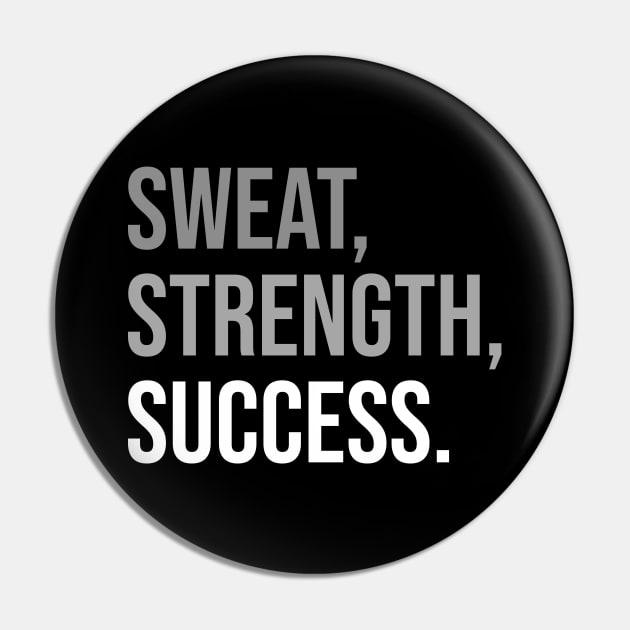The image features a minimalistic, powerful black circular object, possibly a button or tag, set against a contrasting light gray background. Displayed prominently within the black circle are the words "SWEAT, STRENGTH, SUCCESS." Each word is in bold capitalized letters, with "SWEAT" and "STRENGTH" written in light gray and separated by commas. "SUCCESS," which stands out more prominently in white, is followed by a white period. The black circle shows depth with a reflection on the sides, giving it a three-dimensional appearance. The whole design is sleek and simple, emphasizing the progression to success through sweat and strength.